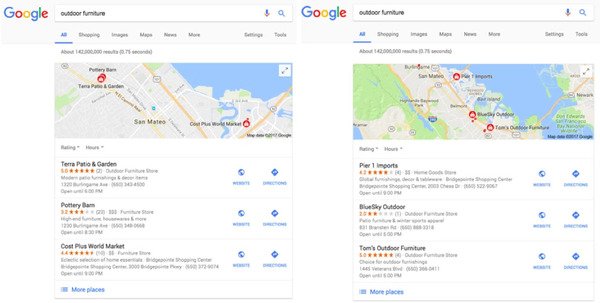The image is a screenshot featuring two different sets of Google search results. On the left side, the search query entered into the Google search bar is "outdoor furniture." The search results prominently displayed include websites such as Terra Patio and Garden, Pottery Barn, and Cost Plus World Market, providing various examples of locations where outdoor furniture can be sourced.

On the right side of the image, the search bar also contains the query "outdoor furniture," continuing with similar types of results. However, due to the cropping or partial display of the screenshot, the detailed listings of the search results on the right are not fully visible, suggesting further examples of retailers or resources for outdoor furniture. This juxtaposition illustrates a comparative look at search results for the same query on Google.